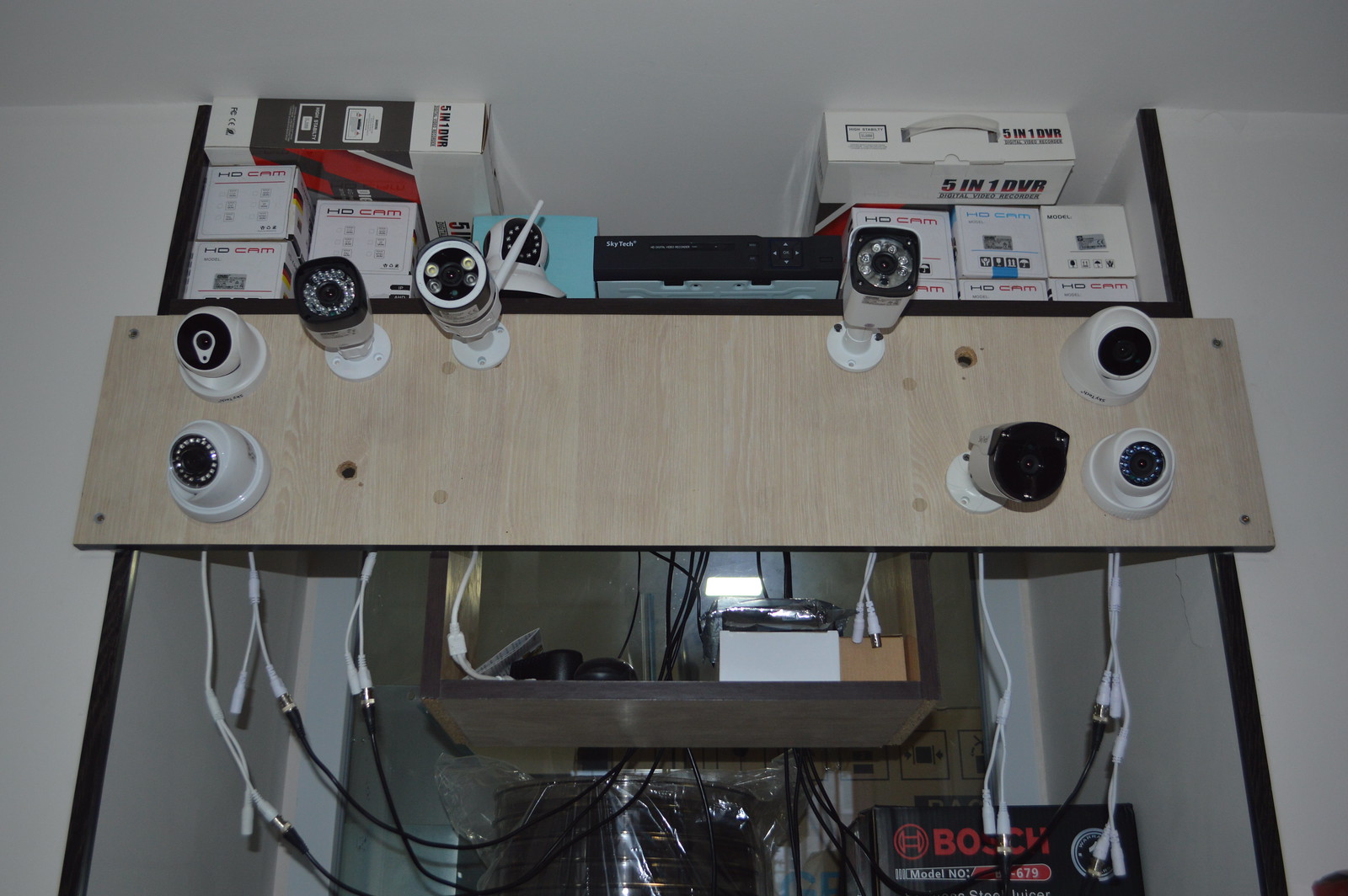In this detailed color photograph, we are looking up at a light brown wooden plank mounted horizontally against a white wall. Attached to this plank are eight brand new outdoor security lights, arranged in a detailed display. On the left of the center, there are four lights, three positioned towards the top and one towards the bottom. Likewise, on the right side, there are four more lights. These lights are primarily circular with white plastic bases and black lenses, although there are some square-shaped ones as well. Below the wooden plank, a tangle of white cords can be seen dangling, ultimately connecting to black cords that lead to a power supply in the background.

Adding to the scene, a translucent box filled with additional equipment, boxes, and more wires is visible beneath the main display. The cords hanging down from the lights on the wooden plank pass through small holes, connecting with the black wires that lead through the translucent box. Above the wooden plank, shelves are holding boxes, presumably packaging for the various lights on display. The setup seems meticulously organized to showcase the functionality and appearance of these state-of-the-art LED security lights, devoid of any visible text or branding in the image.